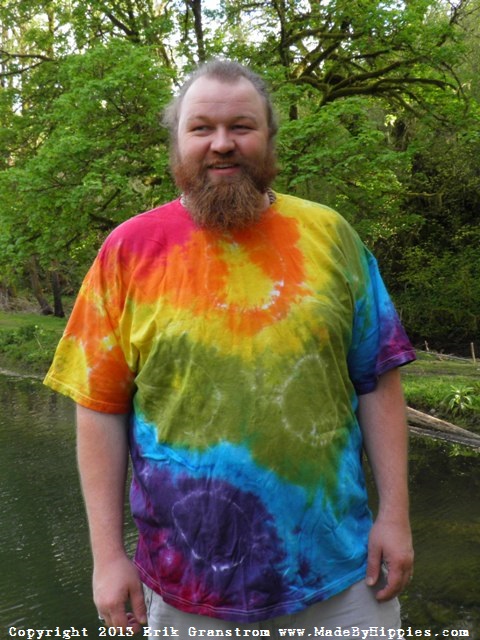The image features a middle-aged white man, likely in his 40s, who has a receding hairline and short, grayish-brown hair. His facial hair includes a scraggly brown beard and mustache. He appears somewhat overweight and is dressed in a vibrant, tie-dye t-shirt that transitions through a spectrum of colors from red at the top to purple at the bottom, incorporating orange, yellow, green, light blue, and dark blue. The t-shirt also has faint white circular patterns amidst the colorful splotches. Although only the tops of his white khaki-like pants are visible, the man stands facing forward while his gaze is directed off to the left. The setting is outdoors in a sunny, open natural area, with a river or pond reflecting greenish water in the background, surrounded by lush grass and numerous tall trees with dense green foliage. At the bottom of the image, white text reads, “Copyright 2013, Eric Granstrom, www.madebyhippies.com.”